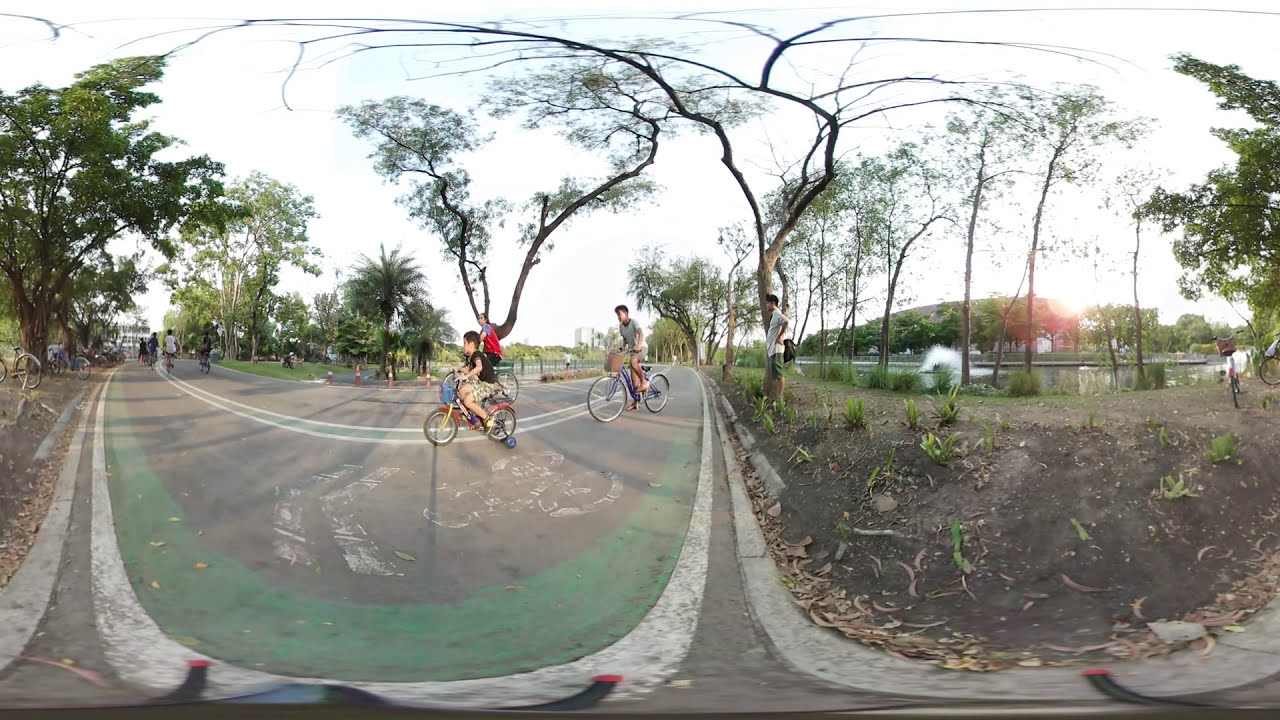This image captures a vibrant, outdoor daytime scene with a fisheye, wide-angle perspective giving a slightly distorted, circular appearance. The primary focus is on a road dedicated to biking, distinguished by noticeable green and white markings that separate the traffic lanes. Multiple people, including children, are riding bicycles on this path. At the forefront is a young boy, around six to seven years old, wearing a black shirt and camel shorts, pedaling a small 20-inch bike with training wheels. Behind him, an older boy, roughly 12 or 13, is on a regular bicycle equipped with a basket. Further back, a child in a red vest over a blue shirt is also biking.

Surrounding the bike path are several green-leaved trees, indicating a lush, park-like environment. On the right side of the image, in the distance, a tree line leads to a large rectangular building with a gray roof. Closer to the foreground, beside this tree line, is a serene pond featuring a prominent water fountain spraying upward, creating a picturesque focal point. The sky above is a dull light gray, yet the sun is peeking through, casting light on the scene despite scattered clouds. A person wearing green shorts is standing by the roadside near the curbs, adding a human element to the lively outdoor setting.